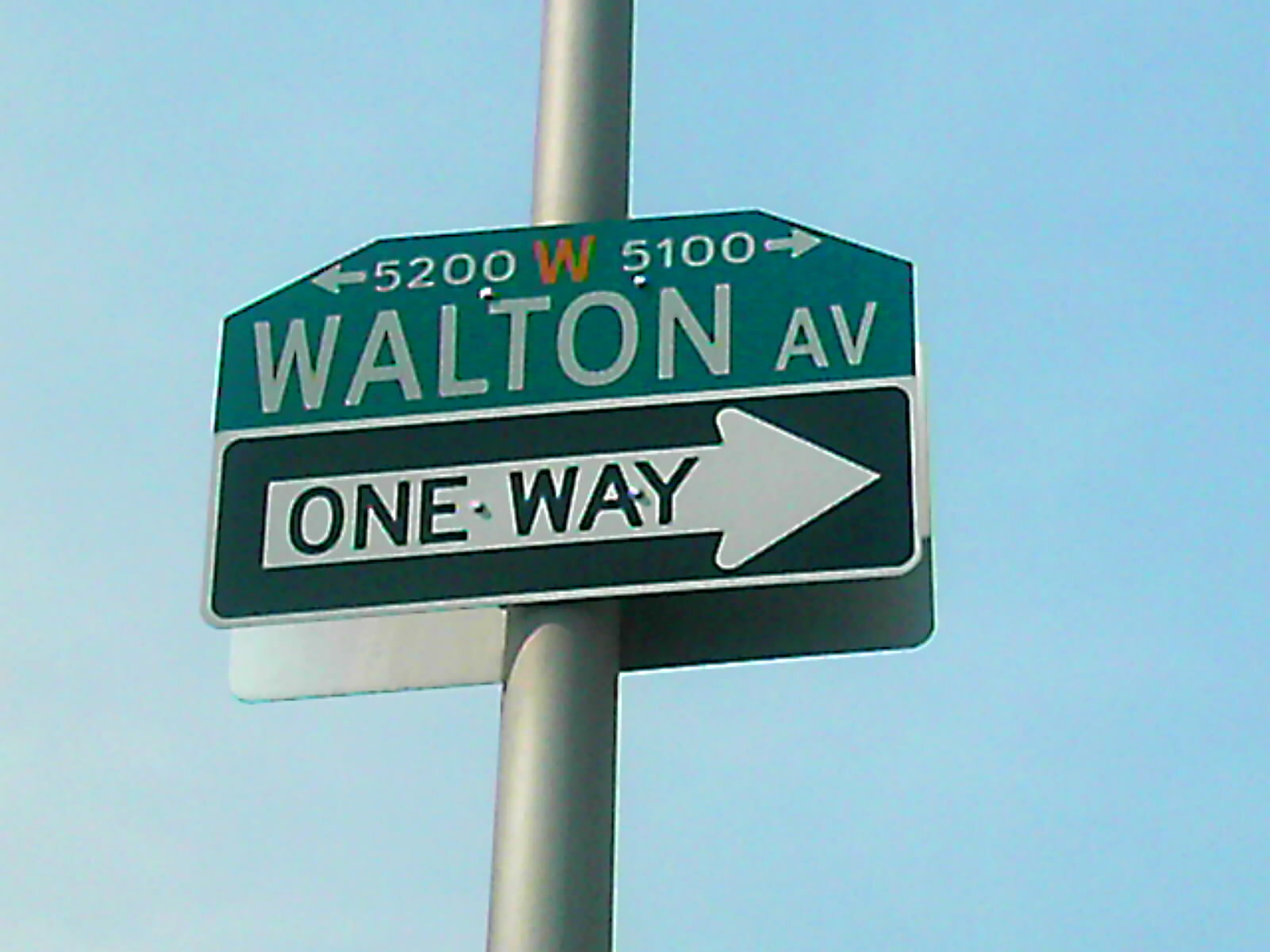This is an extreme close-up photograph of a street sign set against a clear, bright, cloudless light blue sky. Central to the image is a tall, silver metal pole that stretches from the bottom to the top of the frame. Affixed to this pole are two distinct street signs. The top sign features a green background with a left-pointing arrow labeled "5200," an orange "W," and a right-pointing arrow labeled "5100," with the text "Walton Avenue" prominently displayed in bold white letters beneath the arrows. The shape of this sign is somewhat rectangular with an arched top. Below it, there's a One Way sign, which is black with a white arrow and border, containing black text that says "One Way" pointing to the right. The back of another sign is visible behind the One Way sign, revealing its silver color. This detail-rich image vividly captures the clear, beautiful day and the functional design of urban street signage.